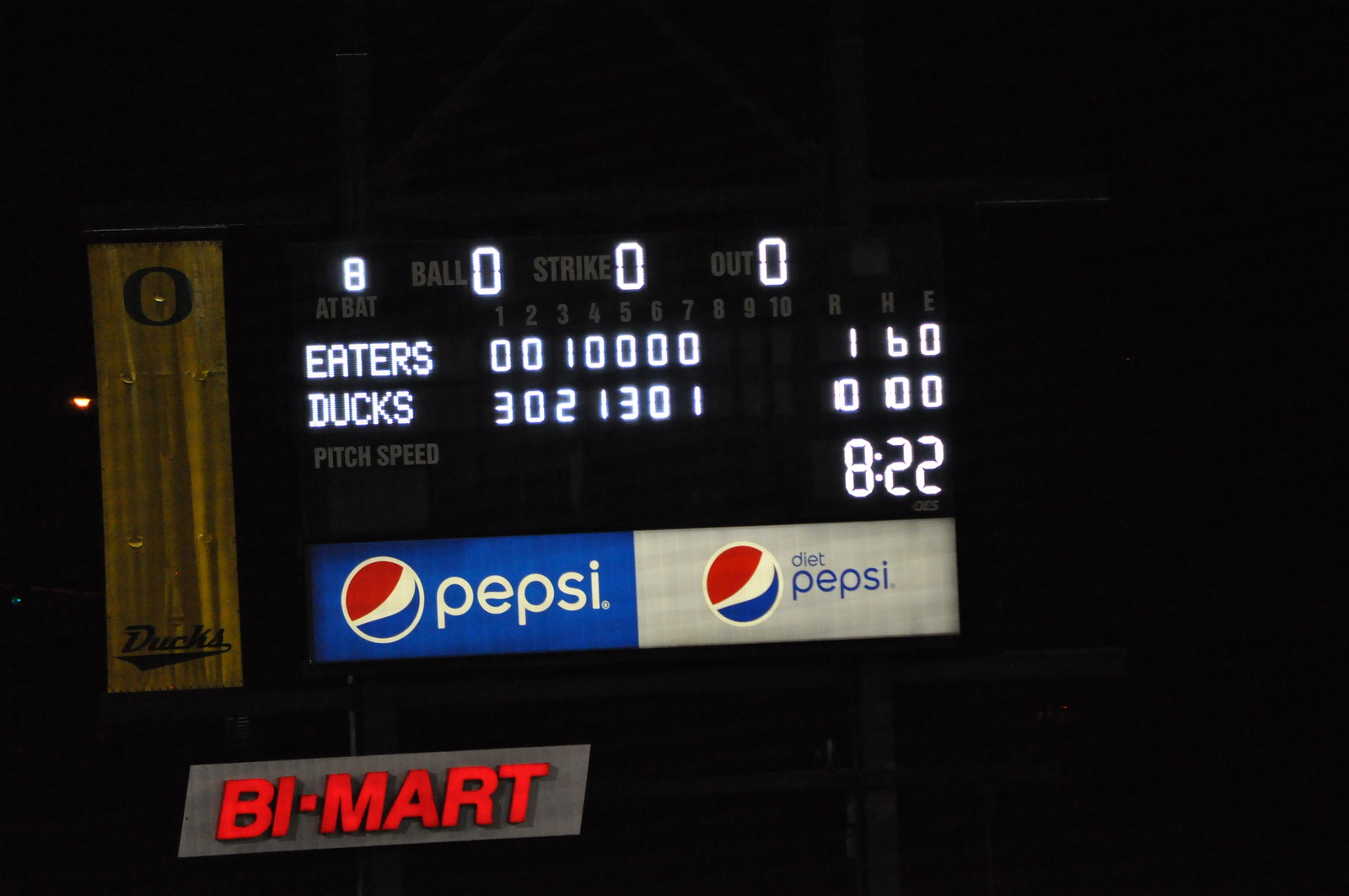This nighttime photograph captures a detailed view of a baseball game scoreboard at a sports facility. The scoreboard lists the competing teams: the Eaters and the Ducks. The Ducks are currently leading with a score of 10-1 in the bottom of the seventh inning. The scoreboard includes details such as a ball, a strike, and an out, along with an unlit pitch speed section that is still readable. The time displayed is 8:22. Prominent sponsorship is evident with the Pepsi logo on the left and the Diet Pepsi logo on the right. Additionally, there is an illuminated "Bi-Mart" sign with red lettering on a gray background at the bottom. A rolled-down vertical banner displaying the word "Ducks" in yellow and black is also visible, although it is not illuminated and harder to see.